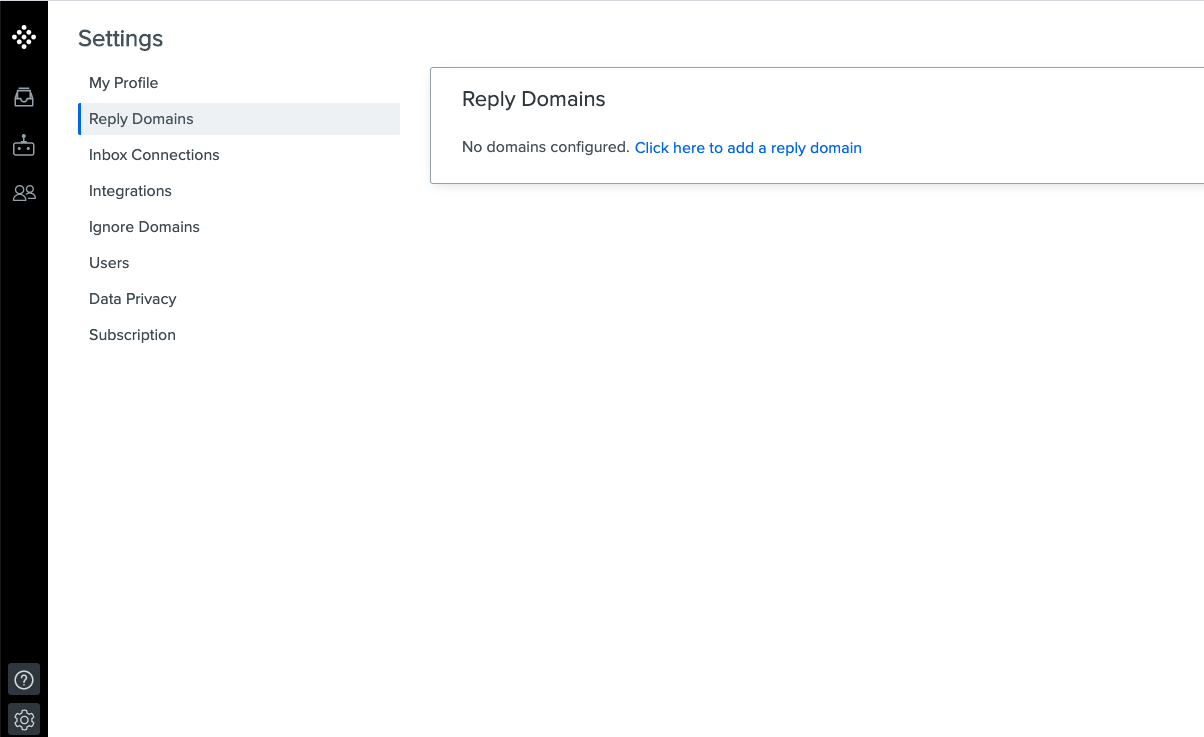The image appears to be a screenshot of a settings page from a web application. The layout is primarily a white background with a sidebar on the left. At the top of the sidebar, the word "Settings" is prominently displayed. Below this, a vertical list includes the following menu items: "My Profile," "Reply Domains," "Inbox Connections," "Integrations," "Ignore Domains," "User," "Data Privacy," and "Subscriptions."

"Reply Domains" is highlighted with a blue line next to it, indicating it as the currently selected option. There is a gray rectangle adjacent to this menu item. Within this section, there's a message stating "No Domains Configured. Click here to add a reply domain," where the actionable "Click here to add a reply domain" text is colored in blue, distinguishing it from the rest of the black text.

The gray rectangle is bordered lightly and appears to be partially cut off on the right side of the image, leaving some elements not fully visible.

On the far left side of the image, there is a small icon consisting of a grid of nine dots arranged in three rows and three columns. Below this, there are additional icons: one looks like a square resembling a Reddit icon, with two dots and an antenna, and next to it are two icons representing people.